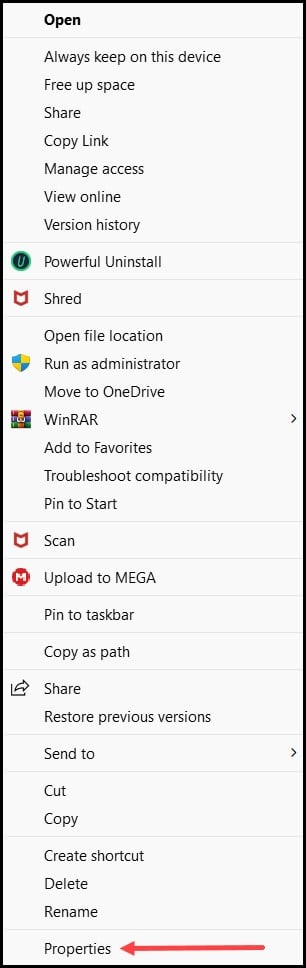The image depicts a standard right-click context menu from a version of Microsoft Windows, most likely Windows 10. The menu presents a wide range of options for managing files, including: 

- Open
- Always keep on this device (OneDrive)
- Open file location
- Run as administrator
- Look to OneDrive
- WinRAR (assumed compression tool integration)
- Add to favorites
- Publish to compatibility
- Start scan
- Upload to Mega (cloud storage)
- Send to taskbar
- Copy as cache
- Share
- Restore previous versions
- Send to
- Cut
- Copy
- Create shortcut
- Delete
- Rename

Additionally, 'Properties' appears at the bottom of the list. The context menu provides access to various functionalities, such as file management, administrative actions, and third-party application features. The image likely portrays a typical scenario encountered when right-clicking on a file or folder within the Windows File Explorer.